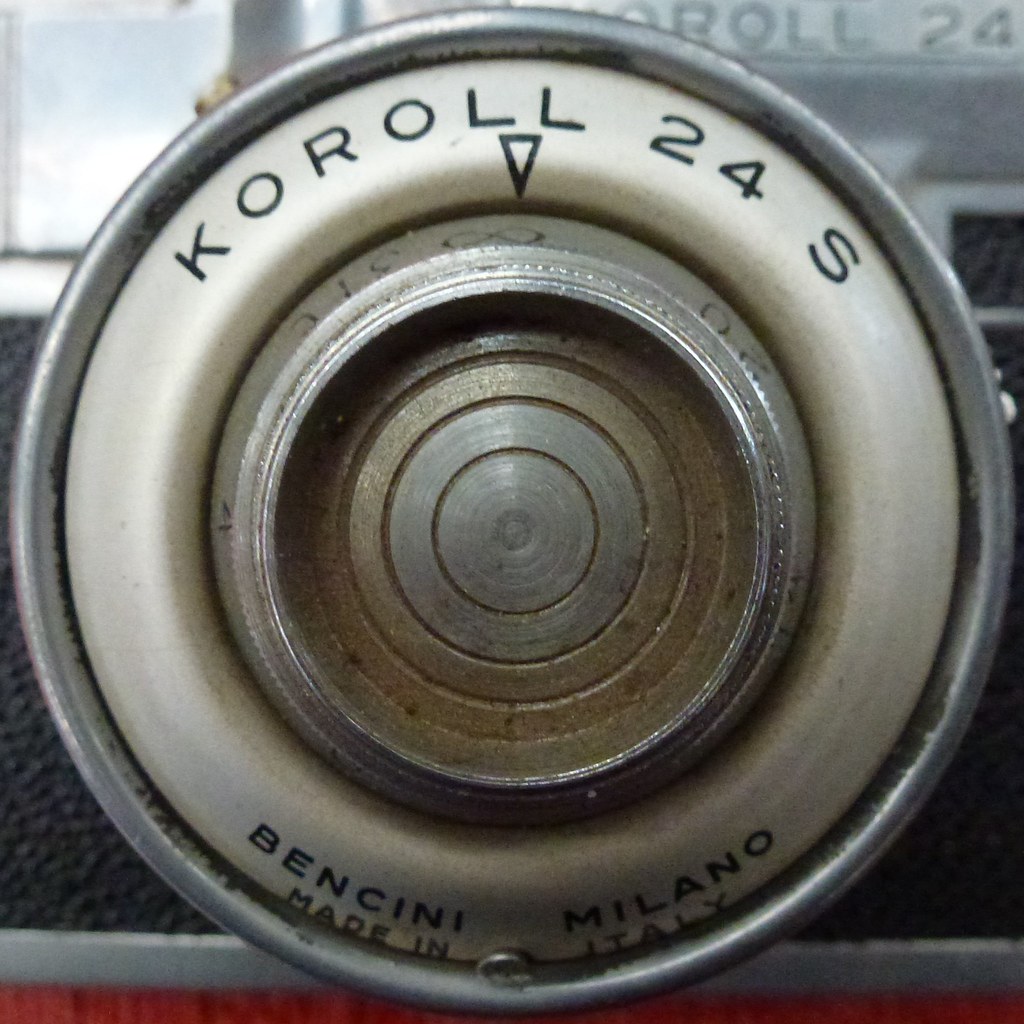The image is an extreme close-up photograph of an aged, metal dial or circular object that is predominantly gray and beige in color, with visible signs of rust and scuff marks. The center of the dial appears older and slightly rusty, surrounded by a white, plastic ring that also shows signs of aging. Prominently, in black lettering, the top of the dial features "Corolle 24S," with a downward-pointing triangle between the last two letters. Below this, it's inscribed with "Benzini Milano, Made in Italy." The object seems to be possibly a hubcap or some functional component, potentially used for unlocking or other mechanical purposes. It is attached to a structure, perhaps a rail or wall, with a metal holder featuring a reddish border visible in the background. The intricate details and aged appearance suggest it has been in use for a considerable time.